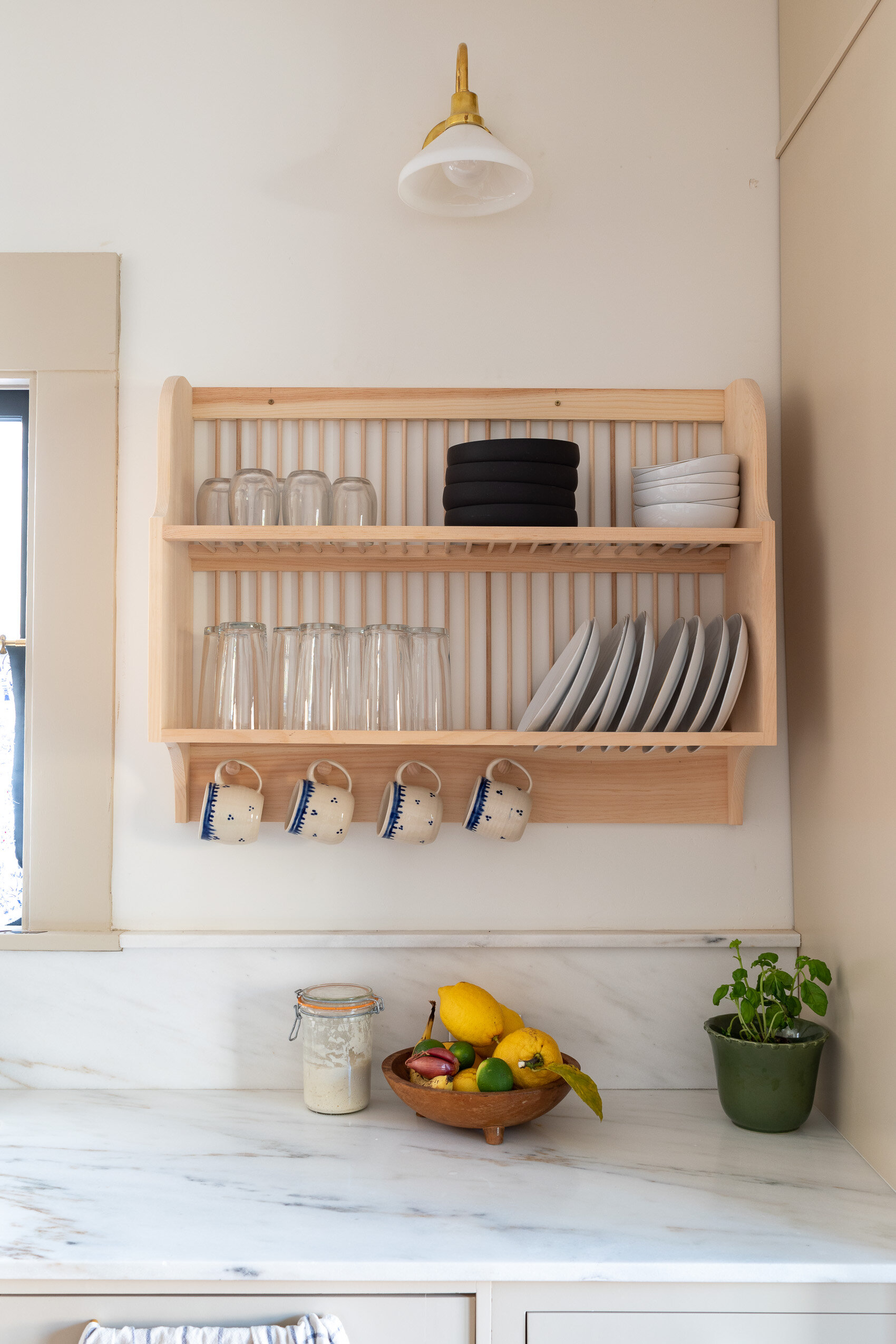The photograph captures a cozy kitchen area inside a home or apartment. The main focus is a wall-mounted shelf unit above a pristine marble countertop. The top shelf of the unit showcases an assortment of white bowls and clear glasses, while the bottom shelf holds larger clear glasses and neatly stacked white dinner plates. Hanging beneath the shelf are four blue and white coffee mugs. Above this arrangement hangs a stylish white and gold lamp, illuminating the space. On the marble counter below, there is a bowl of vibrantly colored fruit, a small potted plant to the right, and a mason jar filled with a white substance. To the left edge of the photo, the faint outline of a window frame is visible. Additionally, a corner of a dish towel peeks out from beneath the countertop, adding a touch of lived-in charm to the scene.